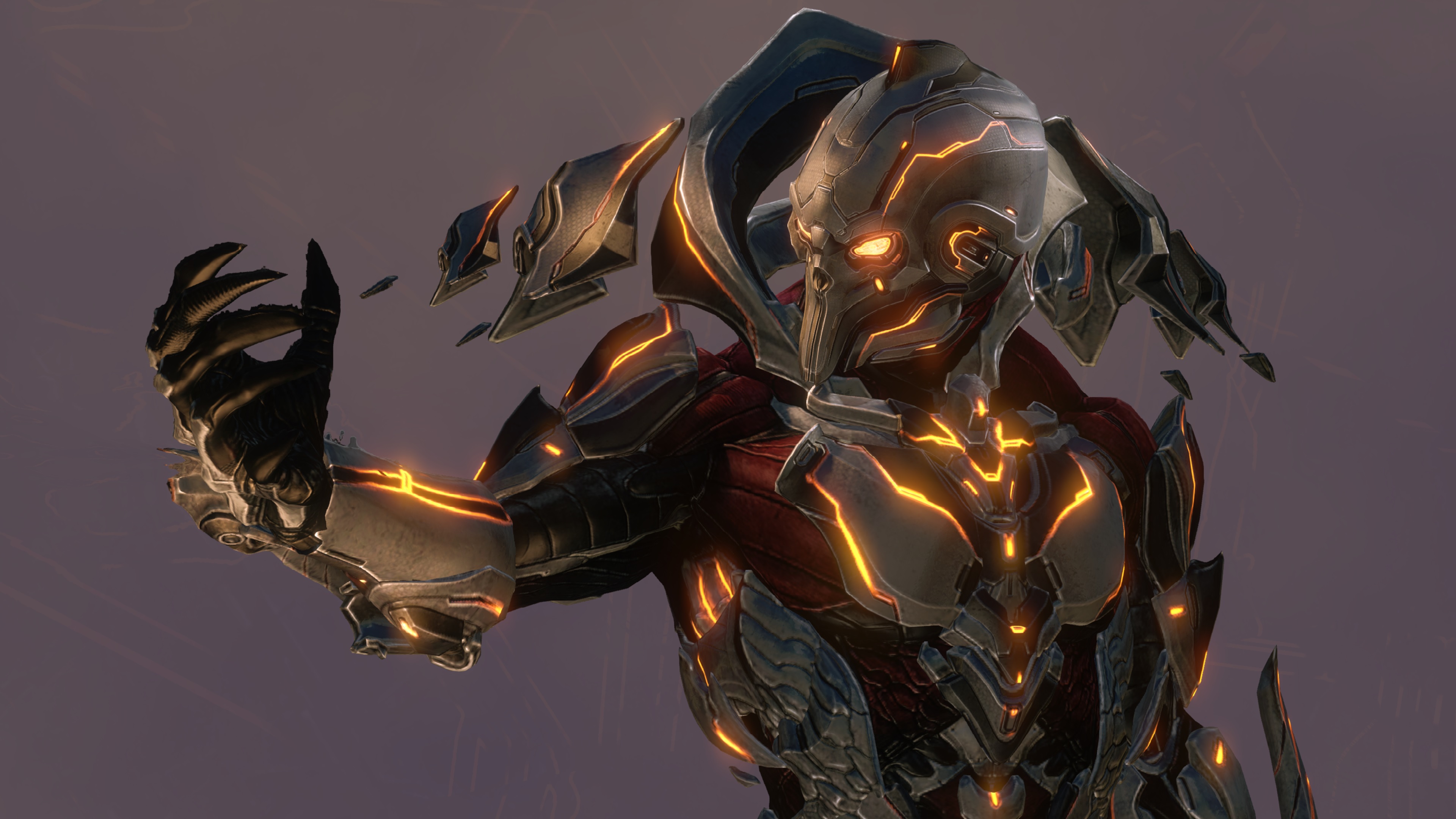In this image, a menacing, futuristic video game character takes center stage, gazing intently from right to left. The character's face resembles a skull, engulfed in golden-yellow-orange flames emitting from its eye sockets, giving the illusion of a helmet. On the left side of this helmet, a small communication device is attached, covering the left ear. The character's body is clad in a tight, red, flesh-like suit with sections of sleek silver metal armor. Highlighting several key areas of the body, glowing amber lights, similar to the ones in its eyes, are embedded around the chest and wrists. The left hand is particularly striking, featuring a gauntlet with long, claw-like nails, adding to the sinister appearance. The overall dark, fearsome aesthetic of this character suggests a villainous role, defined by its skull-like face and the ominous flaming eyes.